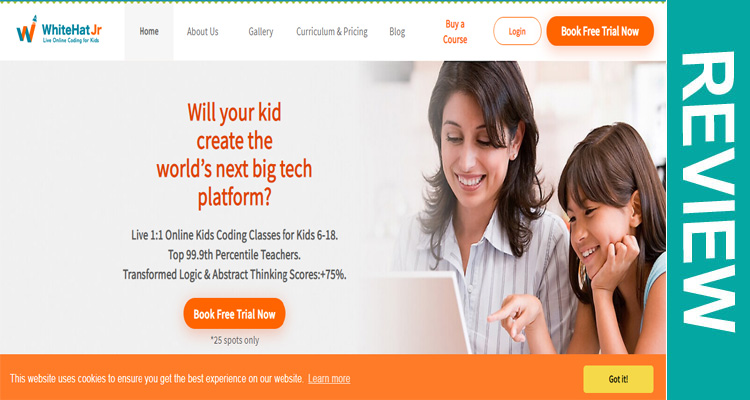The landing page of the White Hat Junior website features a prominent logo in the upper left corner. This logo comprises a stylized "W," with a blue hat perched on the upper right peak. The letter's left-to-right angled segments are highlighted in blue, while the right-to-left segments are colored in orange. Directly beneath the logo, the brand name "White Hat Junior" is displayed, with "Junior" in orange text. Below the brand name, the tagline reads "Live Online Coding for Kids."

Dominating the main portion of the landing page is a large, rectangular message box. It features the headline: "Will Your Kid Create the World's Next Big Tech Platform?" in vivid orange text. Underneath, there is black text stating: "Live 1:1 Online Kids Coding Classes for Kids 6 Through 18. Top 99.9 Percentile Teachers. Transformed Logic and Abstract Thinking Scores by +75%." An orange call-to-action button with the white text "Book Now" is positioned below this message, accompanied by an asterisk indicating "25 spaces left."

The background of this primary section transitions from solid white to gray, blending into an inspirational image of an adult woman with brown hair, dressed in a smart blouse, attentively engaging with a computer screen, laptop, or stack of papers. Beside her is a young girl, using one hand to point to the screen or papers, while her other hand props her chin thoughtfully.

Along the right edge of this section is a teal vertical rectangle containing the word "Review" that is rotated to be read sideways. At the very bottom of the page, a prominent orange banner informs users that "This website uses cookies to ensure you get the best performance." This banner includes a clickable "Learn More" link and a "Got It" button in yellow.

The top of the landing page features a navigation bar with several options: "Home" (currently selected), "About Us," "Gallery," "Curriculum and Pricing," "Blog," and "Bio Course." To the far right of the navigation bar are two action buttons: a white "Login" button and an orange "Book Free Trial Now" button. The entire top section is accentuated by a teal frilled border.